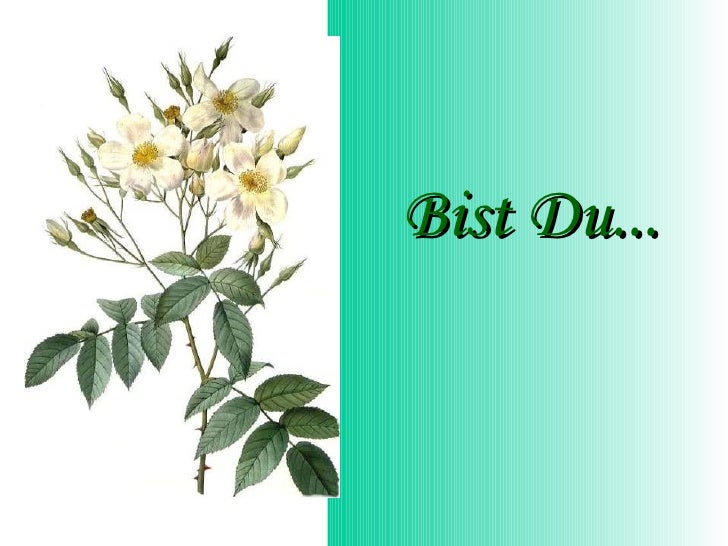The image is divided into two distinct panels. On the left side, there is a detailed, realistic drawing of white flowers with five delicate petals and yellow centers, attached to a thorny branch. Some of the flowers are fully bloomed, while many remain as buds. The flowers are accompanied by muted green leaves that subtly enhance the natural beauty of the scene. 

On the right side, there is an anthropomorphic text design in a script-like dark green font, which reads "bist du..." The background of this panel exhibits a gradient, transitioning from a rich jungle green to a lighter turquoise aqua color that fades into white towards the right edge. The overall layout and elements suggest that the image might serve as the opening slide of a sentimental digital greeting card or presentation, with a likely German phrase that hints at a continuing message. The striations within the gradient and the shadow cast by the text add a tactile sense that complements the delicate nature of the left panel’s floral illustration.